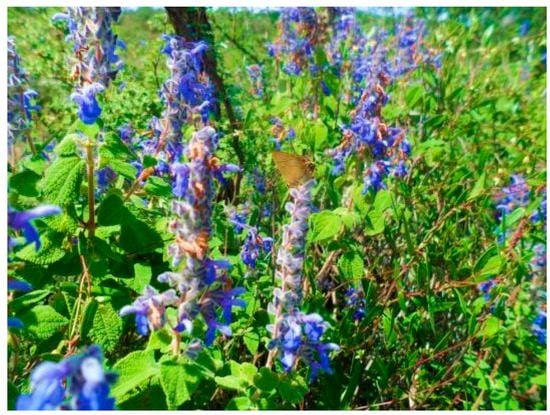This vibrant outdoor color photograph captures an up-close view of a lush, dense area brimming with wild greenery and vibrant purple flowers. The green leaves are thick and intertwined, creating a rich, verdant carpet that is nearly impenetrable. Amidst this sea of green, the flowers stand out on long, elegant stems, adorned with delicate petals that radiate in various shades of bright purple, deep blue, and violet. In full bloom, these flowers sprout along the stems, adding a burst of color that contrasts beautifully with the surrounding foliage. The background reveals a light blue sky visible through small gaps in distant trees. Adding to the scene's dynamic nature, a brown moth or butterfly rests atop one of the flowers. The composition is framed by a mix of green leaves and twigs, focusing attention on the central cluster of flowers, which dominate the field with their vivid hues.